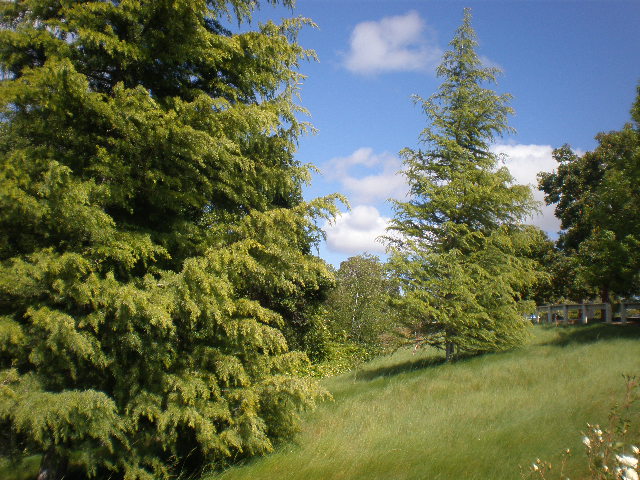The image showcases a picturesque landscape of a sloping grassy hillside under a light blue daytime sky adorned with white and light gray clouds. Dominating the scene, the grassy hill slopes downwards from the higher right side to the lower left side, and is populated by numerous full-bodied pine trees. To the right of the image, a road barrier composed of multiple rounded pillars and a metal railing runs horizontally, marking the edge of the hill. In the bottom right corner, a brown stem adorned with white flowers peeks into the frame. Further in the background, an imposing cedar or spruce tree stands prominently on the left, with a large pine tree positioned behind it. Distantly, a line of large and full trees forms a natural boundary at the back. The setting, devoid of any textual elements, paints a vivid picture with lush greens, natural browns, and the serene blues and whites of the sky.